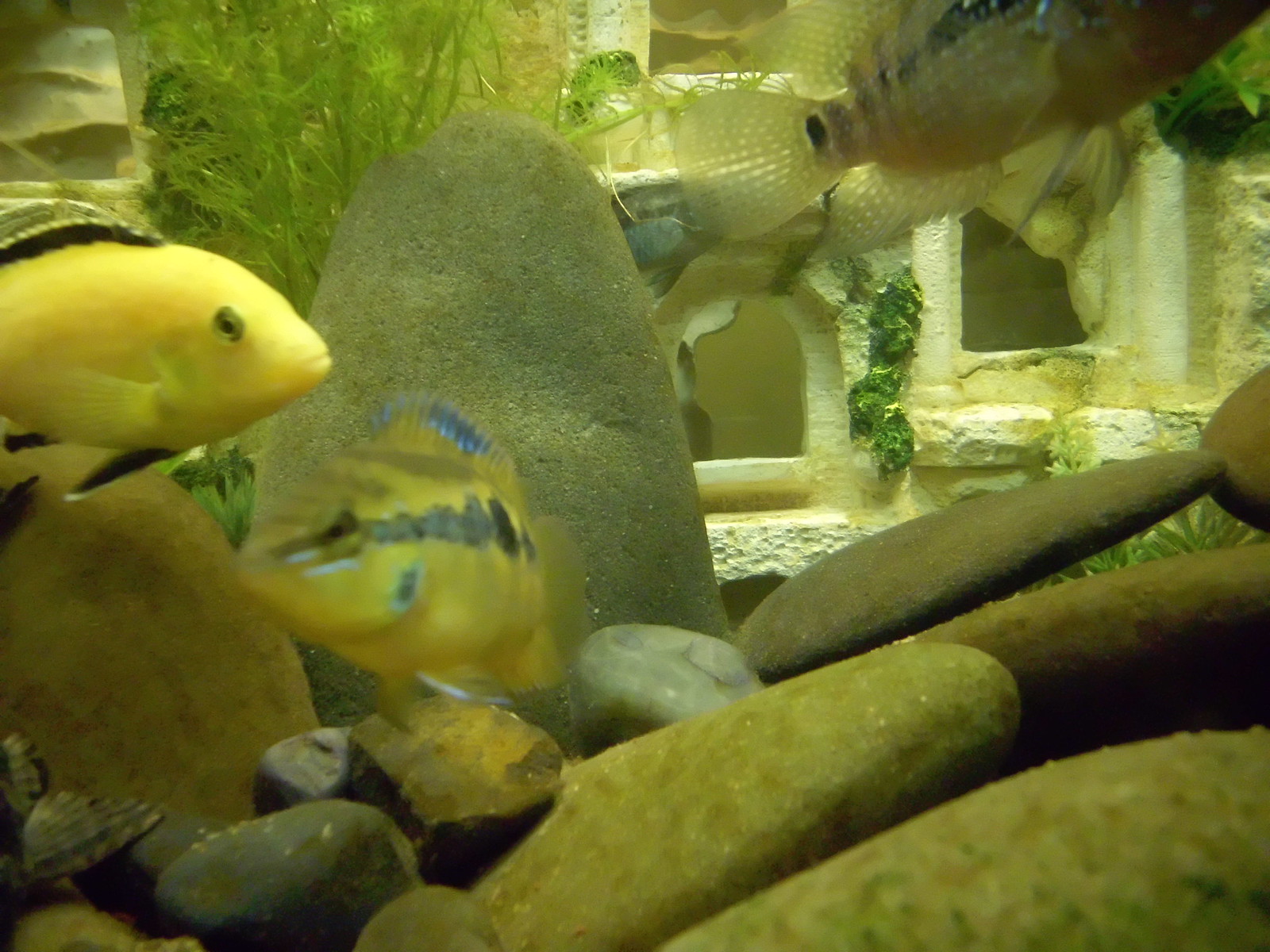This close-up photograph captures an underwater scene inside a rectangular aquarium. The tank's clear glass allows for a vivid view of the aquatic life within. The bottom of the aquarium is lined with smooth brown rocks. Throughout the tank, various water plants add to the natural feel of the habitat. 

In the foreground on the left, a bright yellow fish with a black dorsal fin and a black pectoral fin swims towards the right. Just to the right of this fish, another yellow fish with a striking green stripe along its side moves slightly towards the viewer. The top right corner of the image features a nearly translucent fish with a similar green stripe, as it swims out of the frame. This translucent fish appears to lack pronounced coloration aside from its distinctive stripe. Behind this fish, a decorative element resembling a sandcastle can be seen, adding a whimsical touch to the tank's décor.